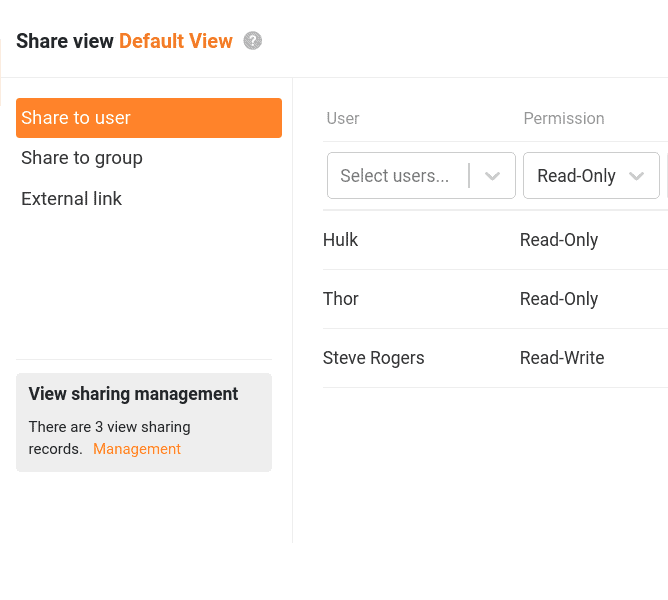**Screenshot of a Browser Interface for Sharing Management**

The image is a screenshot of a browser interface, set against a white background. On the upper section of the interface, there is a navigational text. Part of this text reads "Share View" in black, while another part reads "Default View" in orange, separated by a question mark. 

The left pane is segmented into sections with the following labels:
1. "Share to User" which is highlighted in orange.
2. "Share to Group."
3. "External Link."
   
In the same pane, at the bottom, there is a substantial gap followed by a gray box containing the text "View Sharing Management." Within this box, there are three records labeled under "View Sharing Management," where the word "Management" is highlighted in orange.

The right pane is divided into two columns labeled "User" and "Permission," each with a dropdown box. The dropdown for "User" is labeled "Select Users," and the dropdown for "Permission" is labeled "Read Only." Below these dropdown boxes, there are specific user permissions listed as follows:
- User: Hulk; Permission: Read Only
- User: Thor; Permission: Read Only
- User: Steve Rogers; Permission: Read/Write